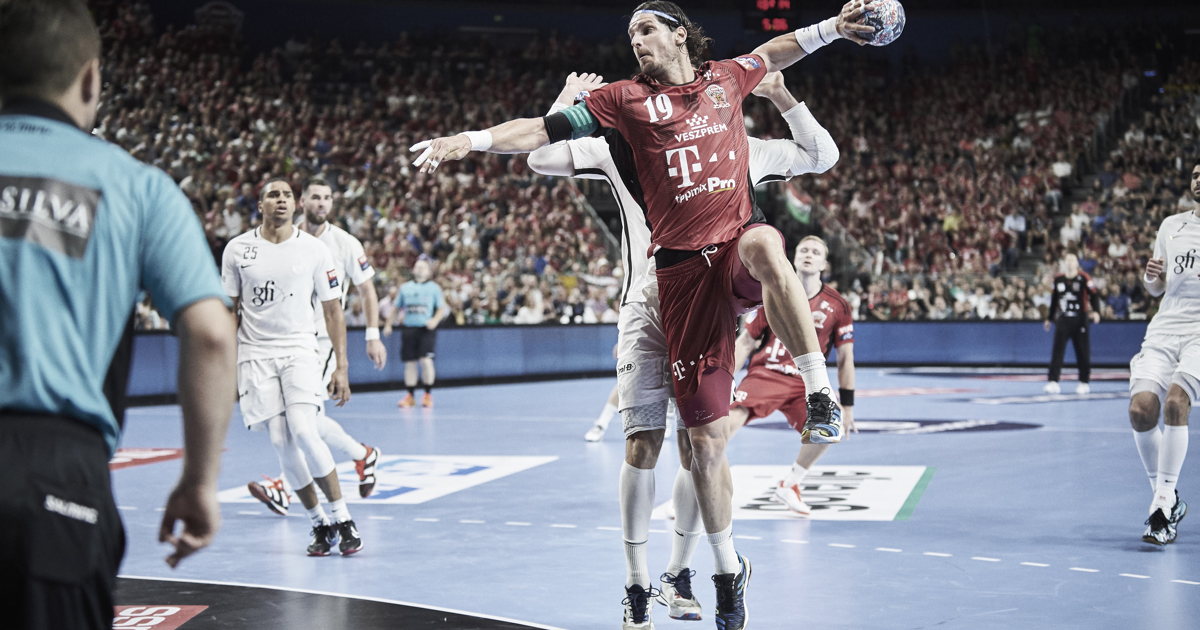This photograph captures an intense moment during a sporting event in a packed indoor arena. The smooth-surfaced, blue court is bustling with action as players in red and white uniforms compete amidst the enthusiastic roars of a full house of spectators. The focal point of the image is a player in a red uniform, adorned with the number 19 and a T-Mobile symbol. He is suspended mid-air, with his left knee raised and his right leg slightly off the ground. 

His left hand grips a small ball, and both arms are outstretched, preparing for a decisive throw. His face, turned to the left, radiates determination. Directly behind him, a player in a white uniform is close, seemingly attempting to block or intercept the play. Other players in both red and white uniforms populate the court, each engrossed in the fast-paced game.

Officials in blue shirts and black pants are strategically positioned around the court, with one notably in the bottom left corner of the frame. In the background, the grandstands are packed with hundreds of spectators, all fixated on the unfolding drama of the game. The event appears to be one of significant importance, possibly an international competition, given the intense atmosphere and the varied languages on the uniforms.